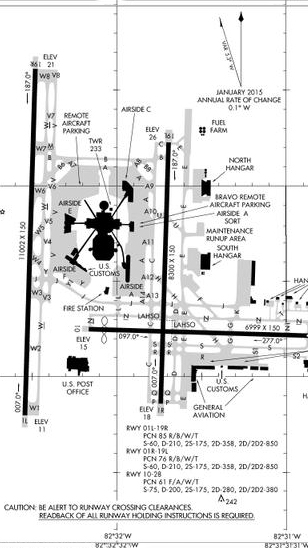This detailed image is a comprehensive map of an airport or airfield, indicated by the various elements and labels displayed. The central area prominently features Airside E, Airside F, and Airside A. Towards the center, there are additional specific locations such as remote aircraft parking and a chopper landing pad with a helicopter icon. Key facilities like U.S. Customs and a U.S. Post Office are clearly marked on the periphery. Consistent with the theme, areas such as the South Hangar, North Hangar, and Maintenance Run-Up Area are identified.

The map is filled with intricate lines moving in multiple directions, intersected by various letter-number combinations like V4 and V3, possibly representing coordinates, distances, or locations of different runways. Along the lines, there are little dashes, enhancing the map's detailed layout. Annotations include important aviation instructions, particularly at the bottom of the map, with a cautionary note reading: "Be alert to runway crossing clearances. Read back of all runway holding instructions is required." The caption also notes that the map references January 2015 as the period for the annual rate of change and includes multiple latitude and longitude readings to aid navigational clarity. Overall, this detailed map layout illustrates the complex organization of an airfield and serves as a vital tool for understanding the specific locations and logistical arrangements of the airport grounds.